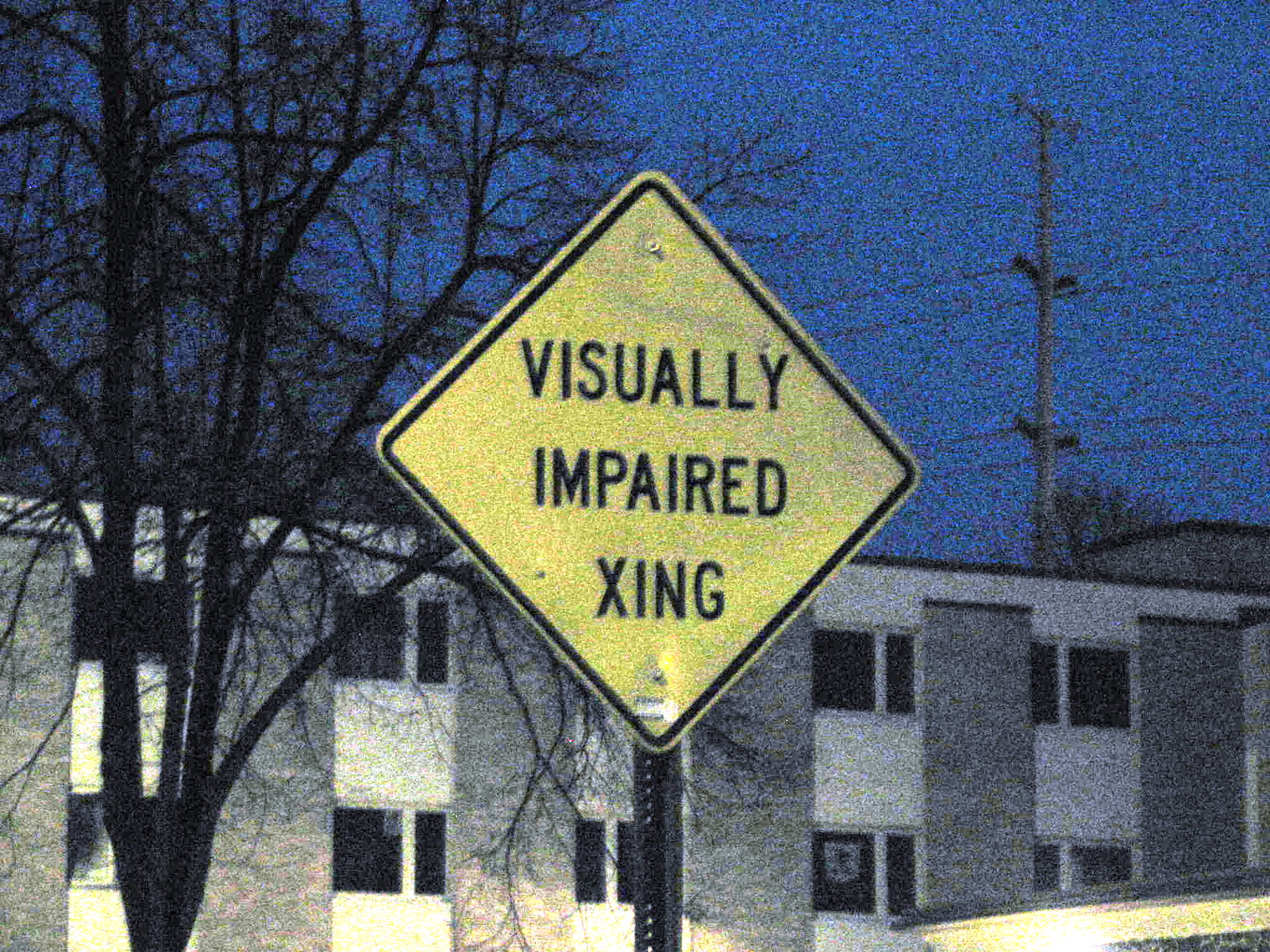The photograph, slightly wider than it is tall, captures a winter scene with a deep blue sky, suggesting twilight either before dawn or after sunset. In the foreground stands a prominent yellow diamond-shaped sign with a black border, centered but slightly tilted. The sign displays "Visually Impaired" on the top two lines and "X-ing" on the bottom line in black text. It is mounted on a black metal pole featuring vertical alignment holes. To the left of the sign is a bare tree, further accentuating the wintry setting. Behind the sign, a symmetrical building, reminiscent of a dormitory or apartment complex, looms with its numerous windows. Additionally, three sets of high-tension electrical lines run to the right of the sign, cutting through the sky. The entire image, slightly pixelated, evokes a serene yet crisp evening or early morning atmosphere.